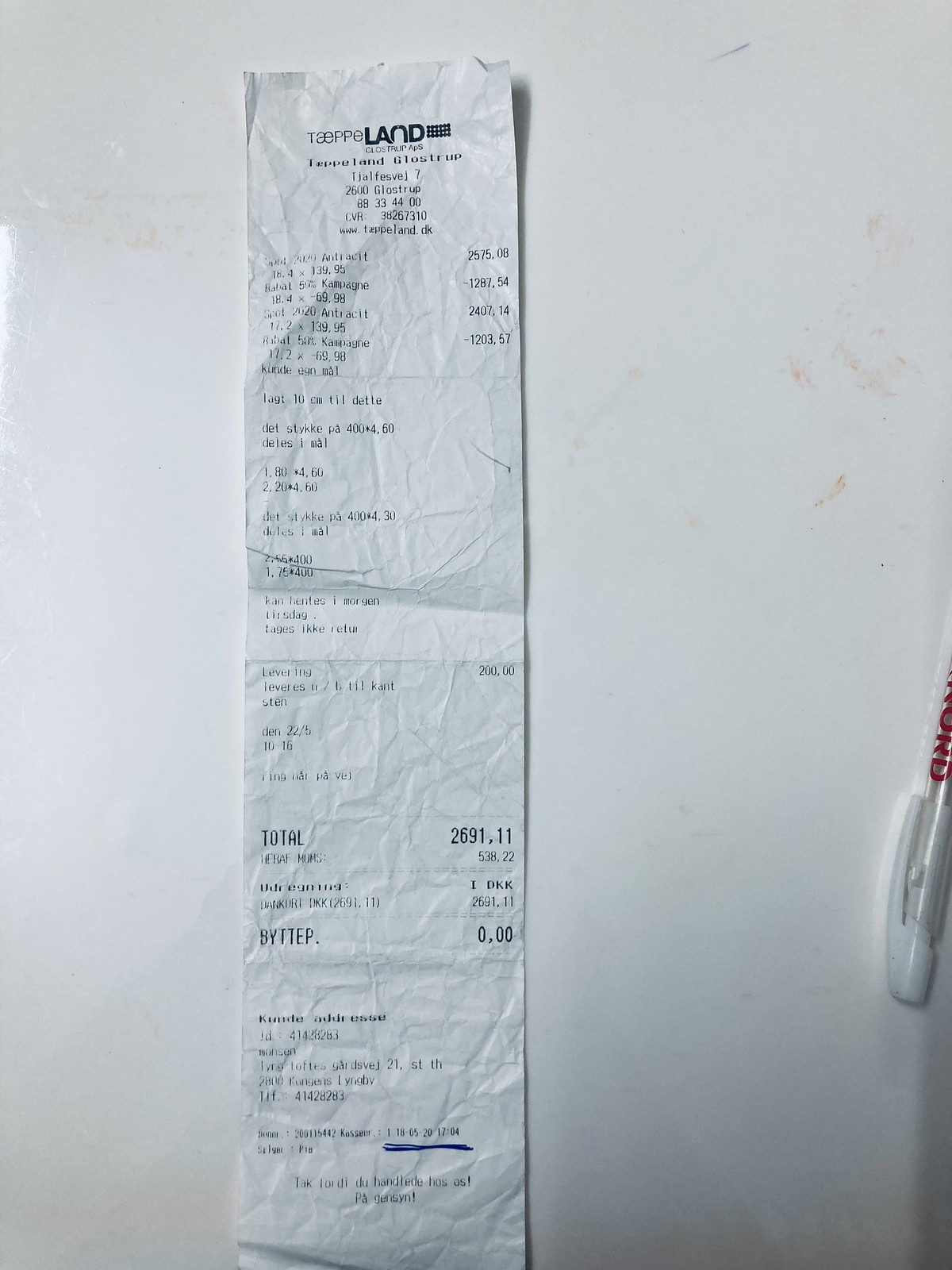This photograph captures an old, heavily wrinkled receipt lying on a white surface, which could be a table or countertop. The receipt extends from the bottom nearly to the top of the image, indicating it is quite lengthy. At the top of the receipt, partial text in black reads "land," though the complete context is unclear. The receipt has been folded multiple times, contributing to its worn appearance, and is riddled with creases and wrinkles. Various numbers and letters are visible on the receipt, but they are mostly indistinct. The total amount at the bottom of the receipt is more legible, showing "2691.111." On the right side of the image, partially out of frame, there is a white pen with red lettering, offering a splash of color amidst the otherwise muted composition. The bottom right corner of the image appears darker, suggesting a shadow or a darker area of the surface.